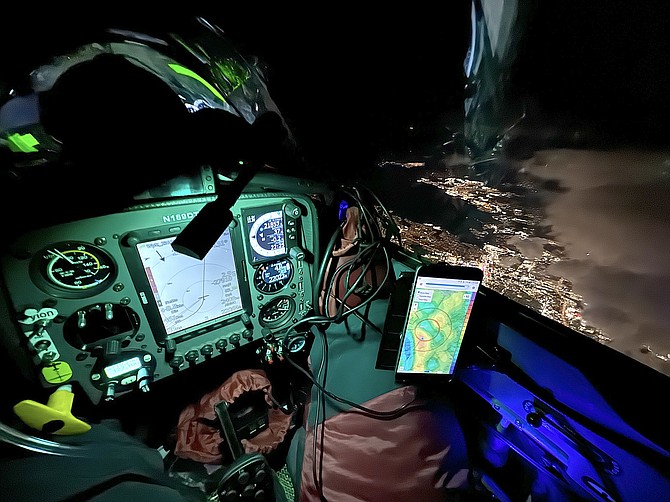The image depicts the interior of an airplane cockpit at night, presumably a jet, from an overhead perspective. The cockpit's dashboard, illuminated with a green light, features an array of controls and instruments, with a noticeable rectangular screen flanked by circular gauges. An iPhone in a holder displaying radar imagery is attached to the panel. Also present are various bags, including a brown and green one, and what appears to be an empty bag possibly resembling a parachute bag, containing an unidentified black object. The cockpit glass reflects the lit-up controls, adding to the complexity of the scene. The view outside reveals the distant ground lights far below, indicating that the aircraft is flying high above the clouds. A blue light can be seen on the right-hand side, contributing to the detailed and multi-faceted visual environment within the cockpit.